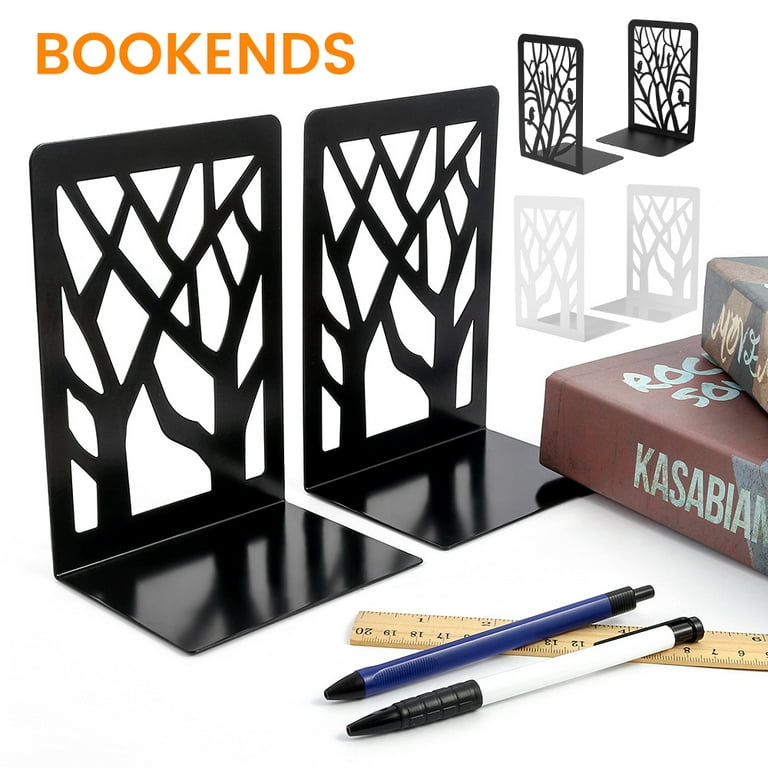This image depicts an advertisement, likely used for a digital marketplace such as Amazon, showcasing a pair of black metal bookends. The top of the image prominently features the word "BOOKENDS" in large orange letters. The bookends are crafted to resemble leafless trees with intricately branching limbs stretching sideways and upward, while the base of each bookend forms solid black rectangles to be placed under the books. The bookends are shown in both black and also available in white or grey. Arranged in the scene, there is a ruler lying in front of the bookends, with a blue and black pen along with a white and black pencil resting on top of it. Two books are stacked horizontally beside the bookends. Another small depiction of the bookends in silhouette form lies just below the main image, further emphasizing the product's design and functionality.